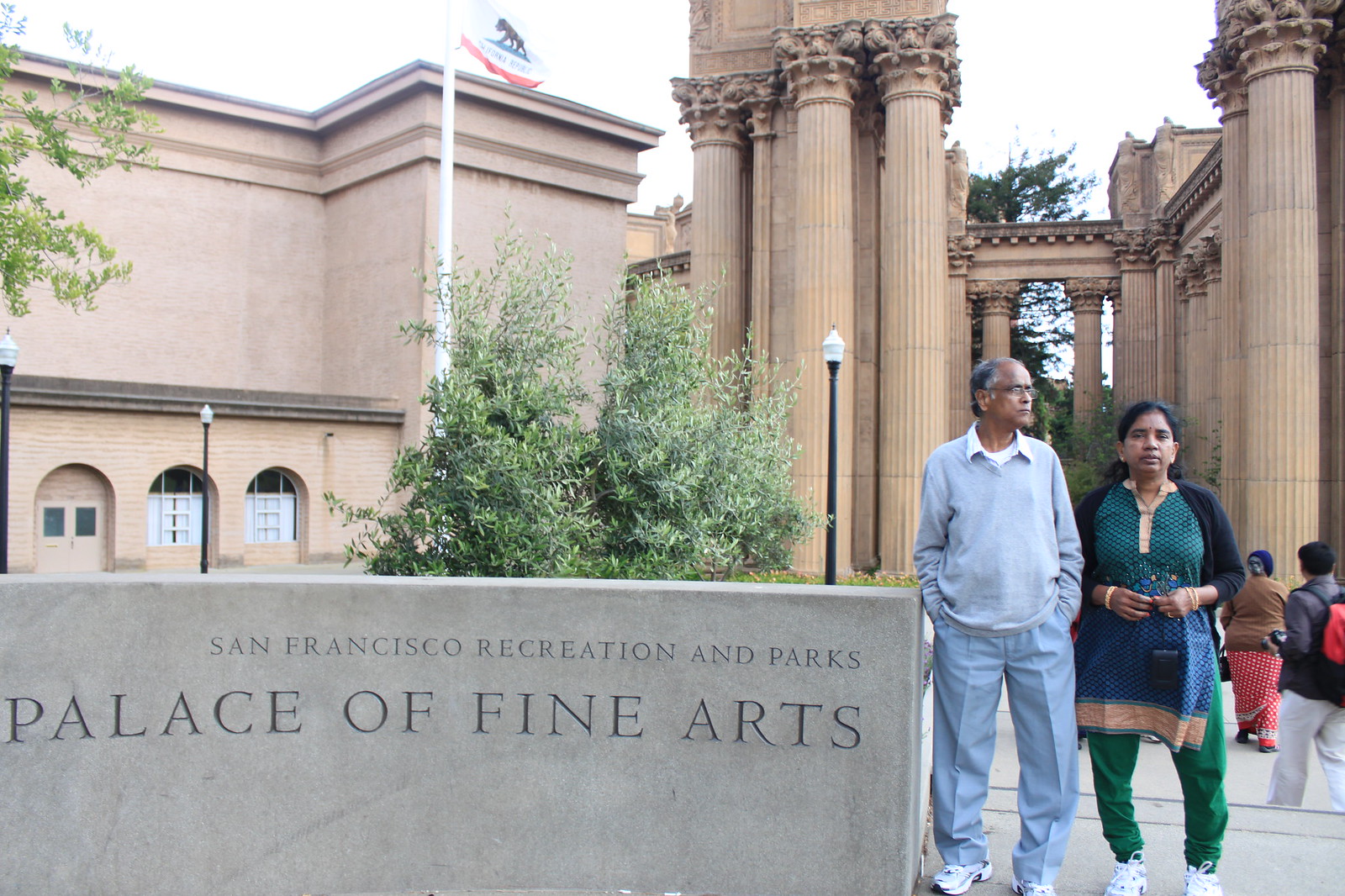In this horizontally aligned rectangular photograph, two people of Indian descent stand in front of a prominent stone wall in the foreground. The wall has an inscription that reads "San Francisco Recreation and Parks" with "Palace of Fine Arts" in larger letters below. On the left, the man, sporting a sweater over a white collared shirt and gray pleated pants, looks off to his right. He has some gray and black hair, wears glasses, and has athletic shoes on. To his right, the woman, with long, black hair tied behind her, wears a blue patterned top over green pants and sneakers. She gazes directly at the camera. Behind them stands a grand building with very tall stone pillars and intricate statues, indicative of the Palace of Fine Arts. Also visible are a couple of trees, bushes, and the California flag with a bear emblem fluttering on a white flagpole with a red stripe. In the lower right corner, the backs of two people walking away from the lens can be seen, and the sky is a bright white backdrop.